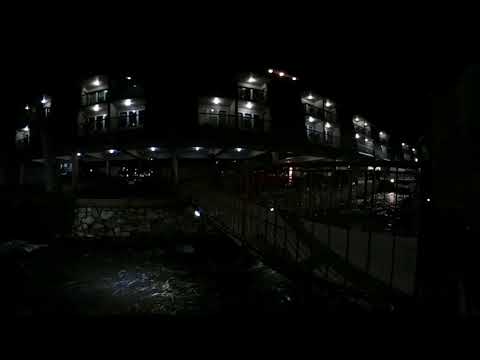This black-and-white nighttime photograph captures a three-story building with a distinctive architectural style, possibly located near Nicosia. The structure, which could be an industrial building, condominium, or hotel, features numerous balconies, each illuminated by a light. The scene is characterized by its darkness, with only the lights on the building and their immediate surroundings being visible. In front of the building, there is a water stream flowing beneath a bridge that leads directly to it. A stone retaining wall runs along the edge of the water, adding to the dockside or riverside atmosphere of the scene. Despite the limited visibility, the photograph effectively highlights the illuminated balconies, contrasting against the otherwise dark environment.